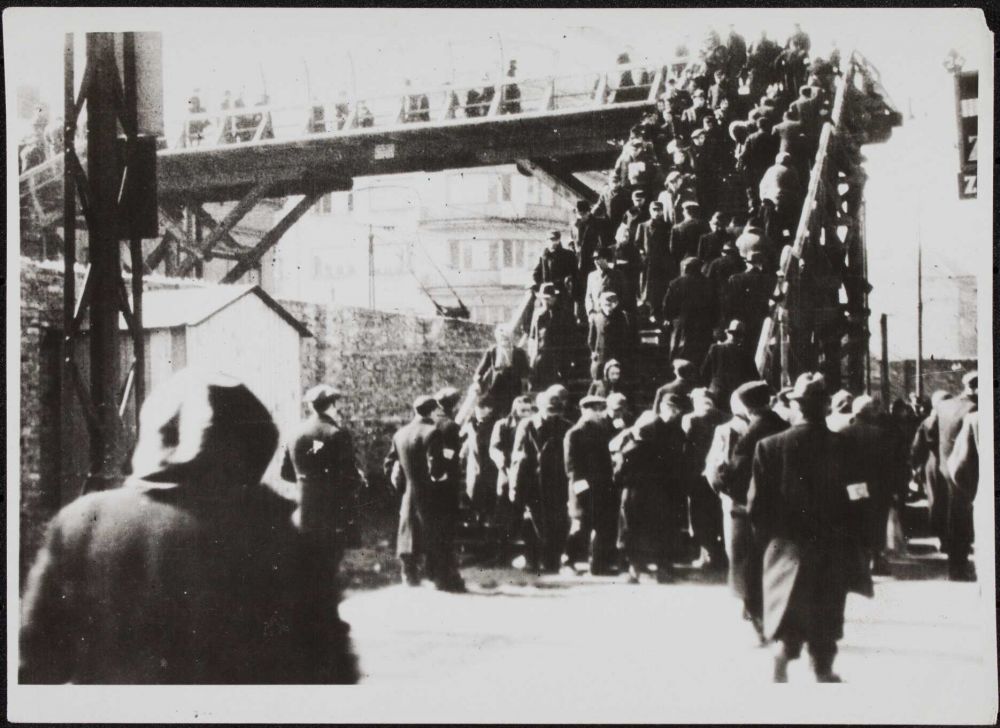This very old, grainy black and white photo captures a bustling industrial scene, likely from the 1930s or 1940s. At its core is a wide, steep iron staircase supported by exposed ironwork, providing access to a catwalk. A large number of men, dressed in period-appropriate attire, are in motion: most are ascending the stairs, some are descending, and a few are gathered at the base. The catwalk appears to stretch across what might be train tracks, hinting at the possibility of a station setting. The photo's left side features iron girders and a tall brick wall, suggesting the structure separates different areas or purposes. Adding to the industrial vibe, a shed-like building stands nearby. The background reveals potential additional details such as an apartment building and an ocean liner, indicating a multifaceted transit hub, where people might be arriving, departing, or meeting others.